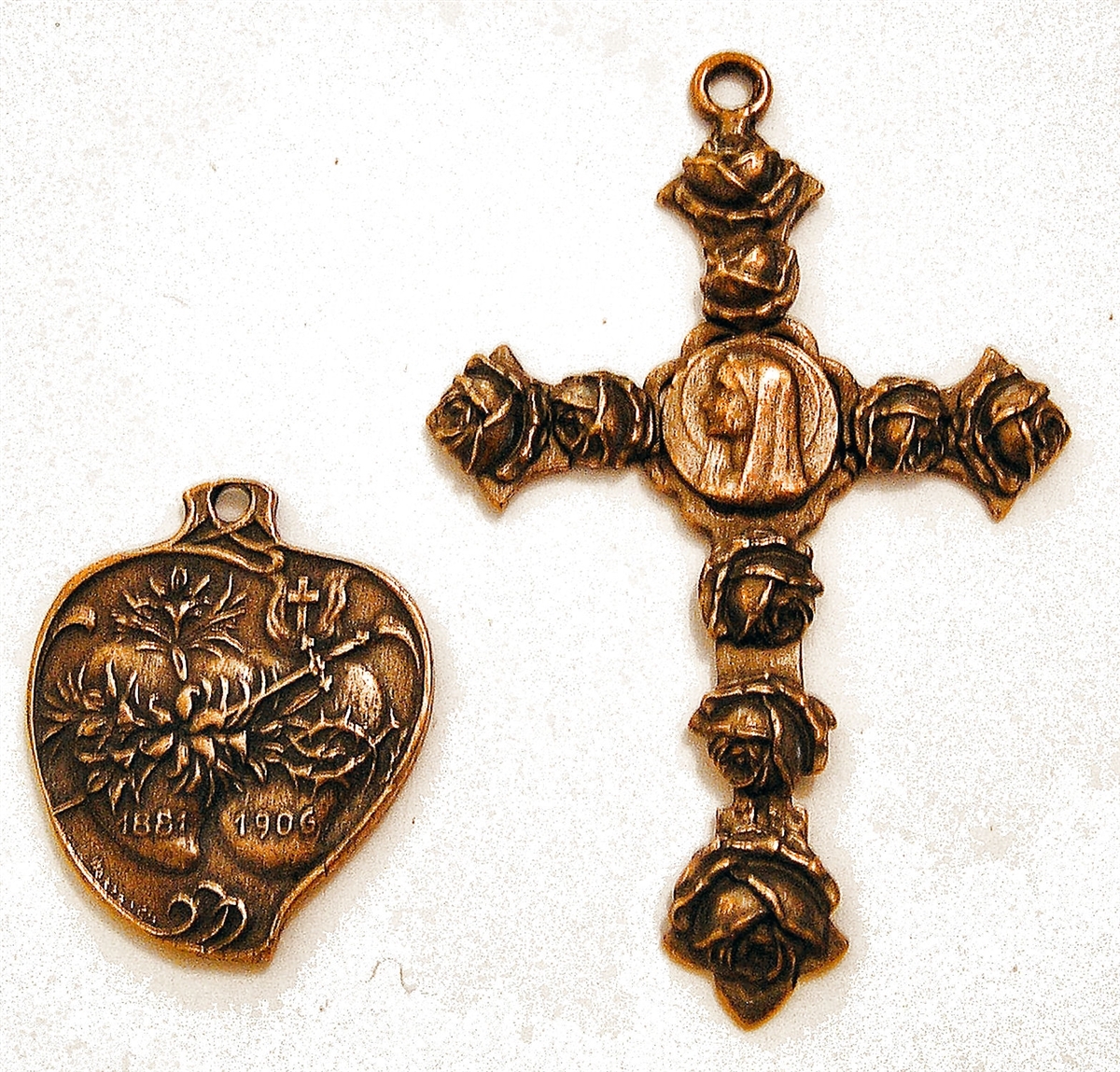In the image, two metalwork pieces rest on a white stone background. The image is somewhat blurry, but the details of the items are discernible. On the bottom left is a heart-shaped or pear-shaped pendant made of bronze-colored metal that varies in shade from darker to lighter spots. This ornate piece features a double heart design, possibly surrounded by thorns, with the years "1881" and "1906" etched on each heart respectively. Above this figure is a small cross. On the right side is a rosary or crucifix, also bronze-colored. It displays a central medallion depicting a woman's face with a shawl over her head. Surrounding the medallion are roses: two on each horizontal arm of the cross and three vertically arranged on the lower part, forming a cross pattern.